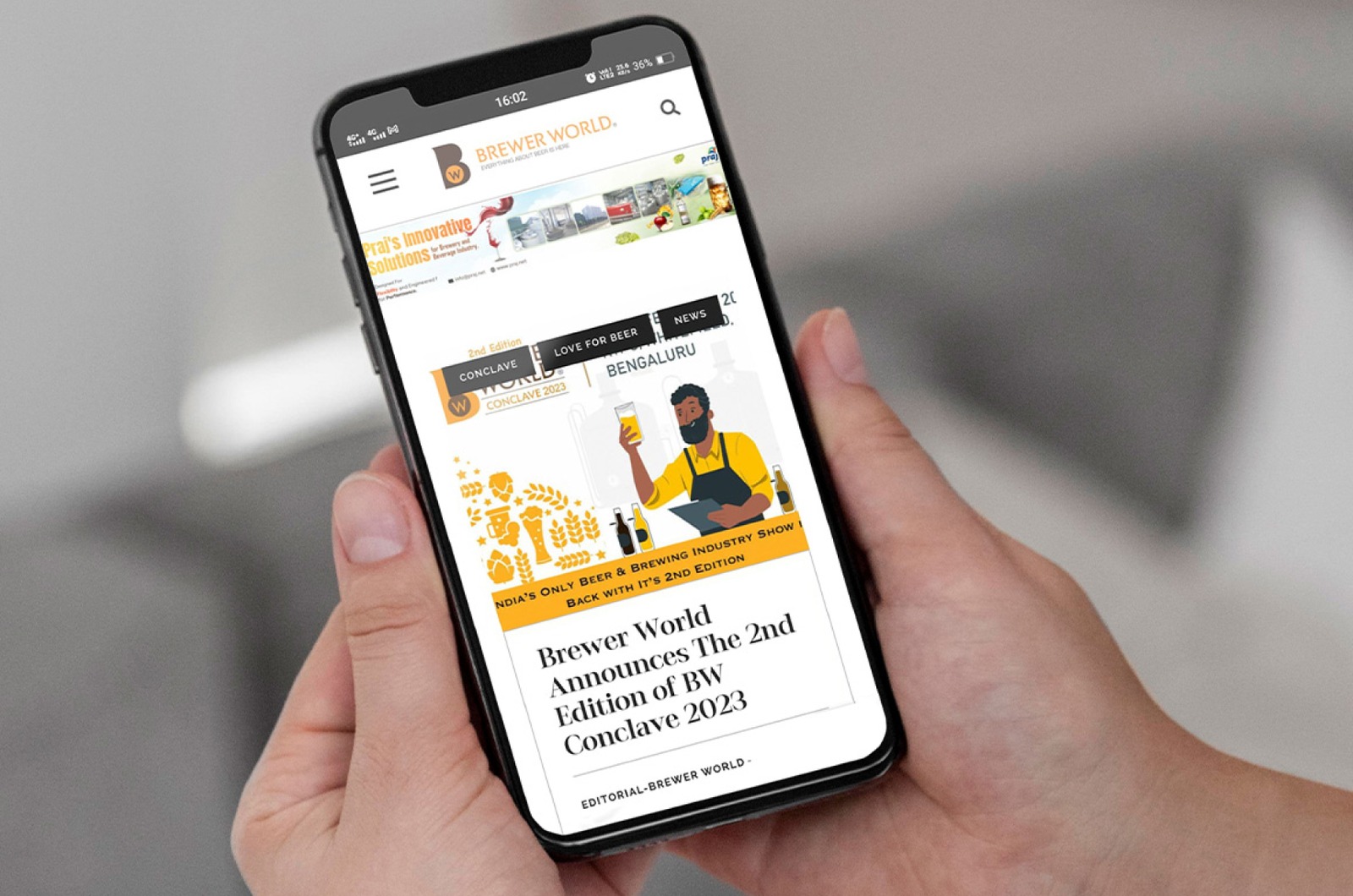A person is holding a black smartphone in their hands, with only parts of their hands visible as they grip the device. The background is blurred and predominantly gray, making it difficult to distinguish any specific details. The visible portion of the phone shows its side buttons, likely for volume control and screen access, and features a display with several elements.

On the top-left corner of the screen, two signal bars are visible, indicating network strength. The top-center displays "1602" in military time, and to the right are several icons, including a clock and two indistinguishable symbols. The battery status shows 36% remaining.

Centered on the screen is the name "Brewer World" accompanied by a prominent logo featuring a large "B" inside a circle alongside a "W". Adjacent to this logo is a three-bar hamburger menu icon. Below these elements is truncated text from an article, including the word "innovative" and what seems to be a media image.

Further down is text that reads "Conclave: Love for beer, news, and black rectangle boxes," accompanied by a cartoon-like illustration of a person holding a beer. The bottom portion of the phone's screen announces: "Brewer World announces the second edition of BW Conclave 2023."